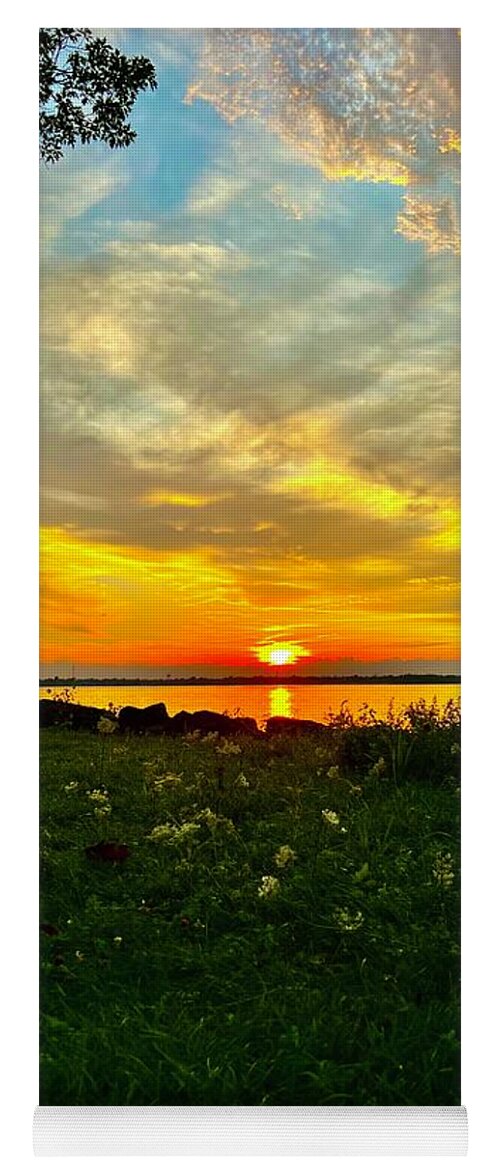The image depicts a long rectangular diamond painting, set upright on a white wooden block, showcasing a highly detailed nature scene. The intricate crosshatch texture of the canvas highlights thousands of individual crystals or colored squares, meticulously forming the vibrant picture. In the foreground, wildflowers and lush grass lead up to a serene lake, where large boulders are visible near the water's edge. The mid ground features the lake itself, reflecting the stunning sunset. The sky is alive with dramatic clouds in shades of red, orange, and yellow, with patches of blue peeking through, creating an awe-inspiring backdrop. Tree branches and leaves frame the scene from the top corners, enhancing the natural beauty. The vivid sunset casts an orange glow, reflecting beautifully off the lake, making the entire painting appear lifelike and captivating.